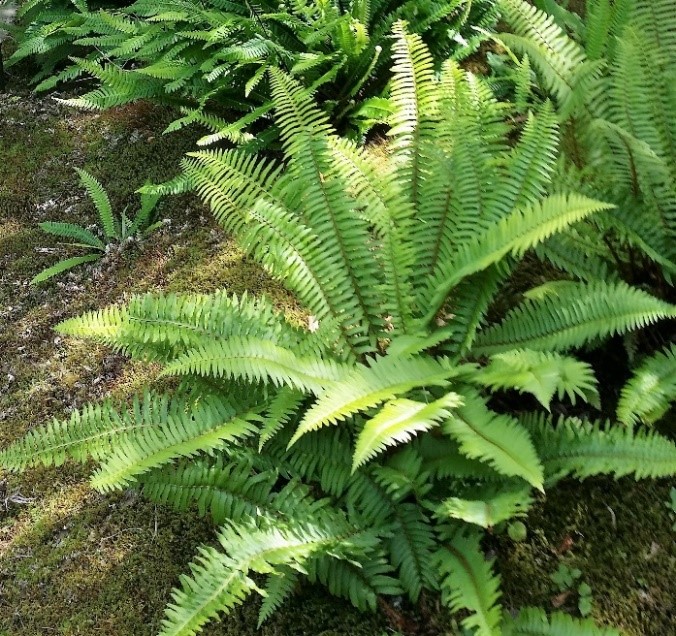The square photograph showcases a lush, forest-like scene with a prominent focus on ferns. These ferns spread across a mossy patch of ground, creating a vibrant, green tapestry. In the foreground, one of the larger ferns dominates the frame, with its long, thin stem and numerous small, oval-shaped leaves that fan out perpendicularly to form an expansive, triangular structure. These leaves are light green and stretch about two to three feet in length. Surrounding this main fern are smaller ones, along with various shrubbery and bushes, all rising from the moss-covered ground. The background features a row of additional ferns, also light green, adding depth to the image. Sunlight filters through the foliage, illuminating the leaves and casting a natural glow on the scene, enriching the lush greenery. Despite a slight motion blur that hints at a casual capture, the photograph beautifully encapsulates the natural beauty and intricate details of the ferns and their mossy habitat.